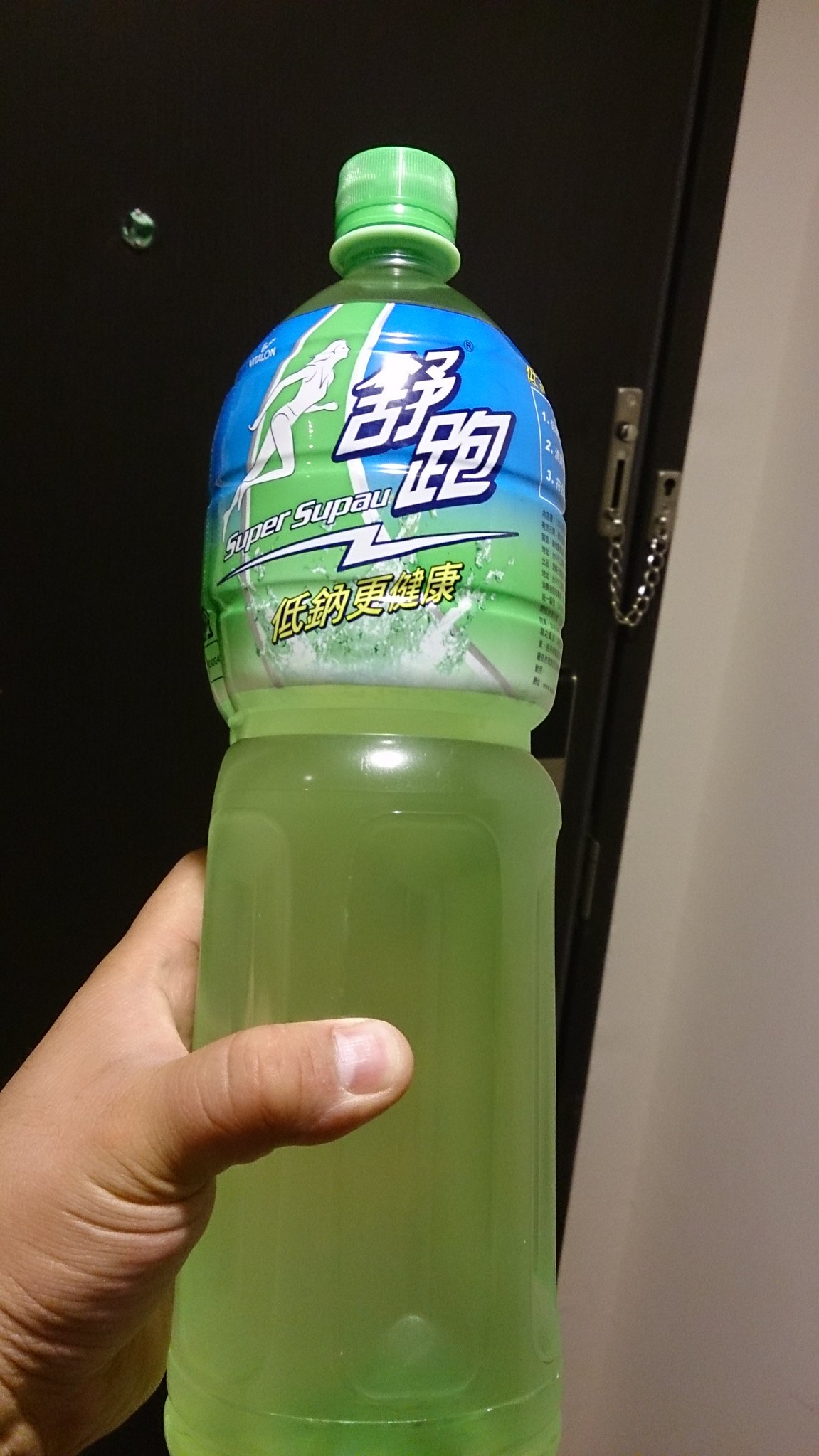A first-person perspective image shows someone holding a large, green-capped plastic bottle containing a green liquid in their left hand. Pronounced Asian lettering, possibly Chinese, adorns the multicolored label, prominently displaying the English words "Super Supau" with a white lightning bolt beneath. The label features vibrant blue and green hues and depicts a running female figure dressed in white, with a green pathway and blue splashes behind her. The background reveals a partially visible left thumb, a black door with a silver chain lock, a large peephole, and a white wall, hinting at a hotel setting. The image appears to be taken indoors with ceiling lighting, likely captured vertically on a cell phone.